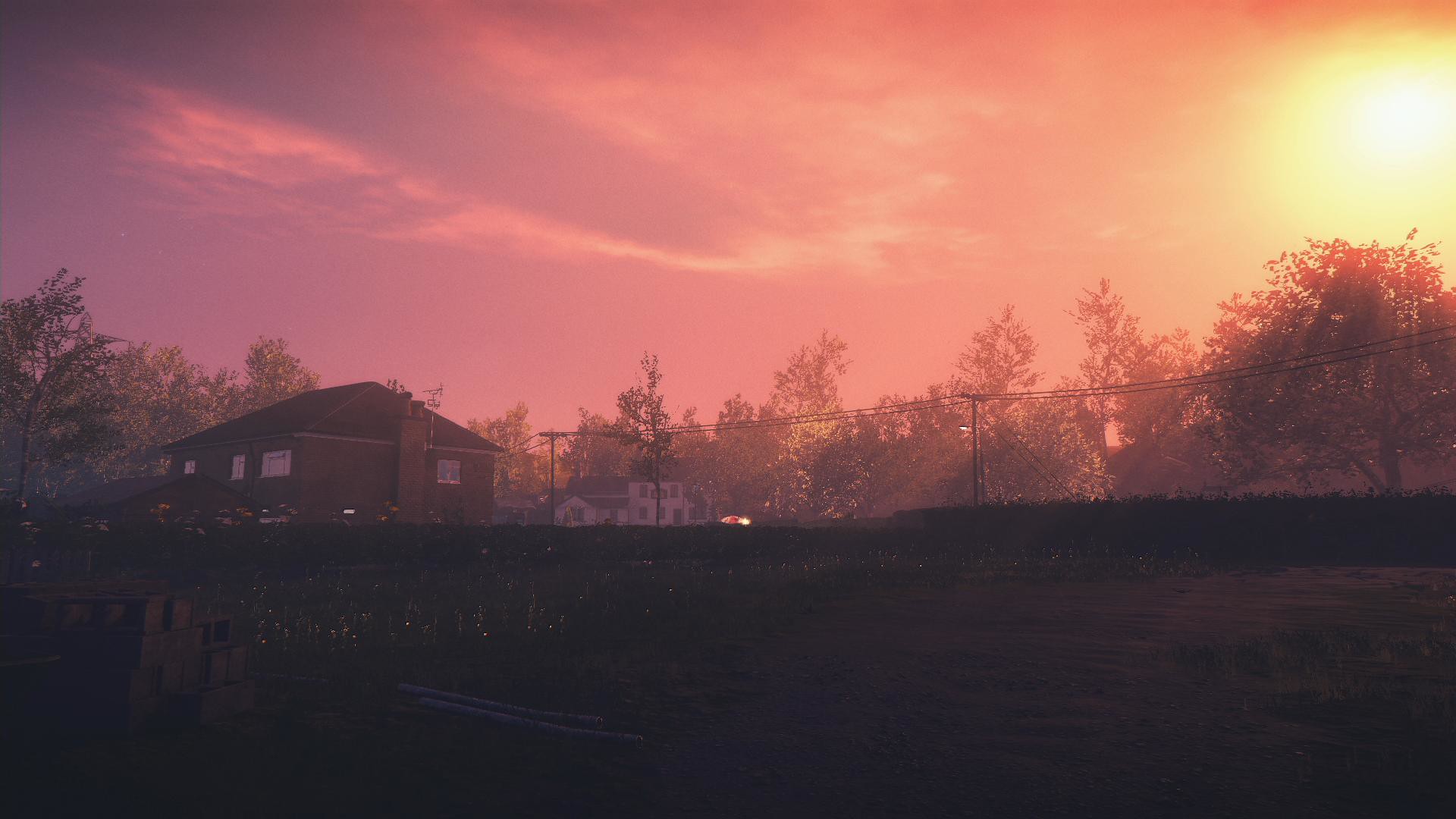This detailed horizontal image, likely from a game or a realistic photograph, captures a residential suburban neighborhood during a vivid sunset. Dominating the left side is a brick house with a black shingled roof and several windows. Power lines stretch across the scene, and trees, glowing with the sunset’s hues, frame the background. In the middle distance, a larger white house stands prominently, hinting at a typical suburban layout. The sky is ablaze with gradients of pinks, purples, oranges, and reds, with the sun positioned at the upper right corner, its white core surrounded by a yellow halo blending seamlessly into the colored clouds. The foreground is marked by a large dark bank, suggesting the photo was taken from a slightly lower vantage point. This twilight scene encapsulates the serene beauty of a suburban sunset, with its play of light and color reflected on the structures and natural elements.